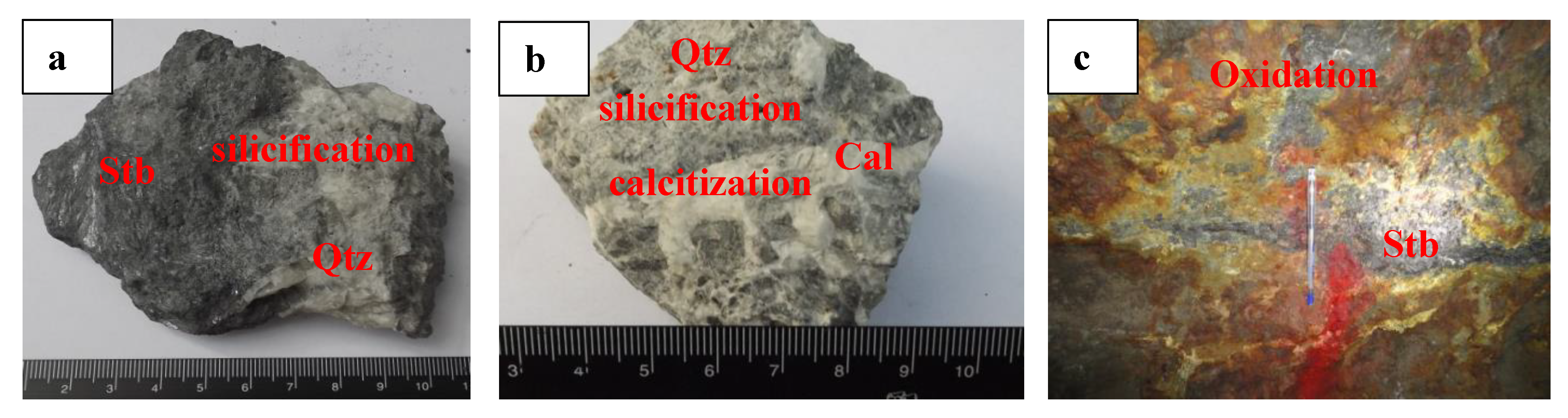The image is a triptych of color photographs arranged side-by-side, each depicting a different rock specimen and labeled A, B, and C from left to right, with black text set into a white rectangle in the top left corner of each image. The leftmost image labeled "A" features a dark gray rock placed next to a black ruler for scale. This rock has red letterings reading "STB" on the left, "solidification" on the right, and "Q-T-Z" beneath "solidification." The middle image, labeled "B," shows a tan-colored rock, with orange text indicating the terms "solidification," "S-I-L-I-C-I-F-I-C-A-T-I-O-N," and "calcification" vertically, and "Q-T-Z" horizontally on the right. The rightmost image, labeled "C," is a close-up of a rock with the word "oxidation" written on it in orange text. Each photograph is roughly the same size and contributes to a detailed, scientifically annotated portrayal of various rock types.